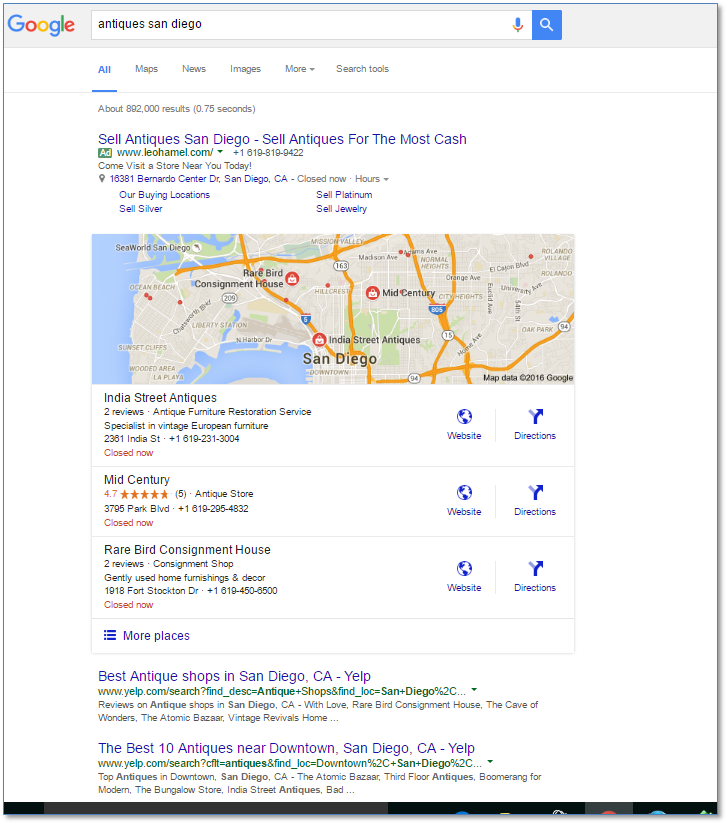A screenshot of a Google search results page is displayed. The user has searched for "Antiques San Diego," and the search yielded approximately 892,000 results in 0.75 seconds. The first visible result is a sponsored ad from Leo Hamel, promoting the sale of antiques with the tagline "Sell Antiques for the most cash" and is linked to www.leohamel.com.

Embedded within the search results is an interactive map of San Diego highlighting three key antique shops: India Street Antiques, Mid-Century, and Rare Bird Consignment House. Each listing includes essential details such as website links, directions, reviews, phone numbers, addresses, and opening hours. Notably, all shops are closed at the time the screenshot was taken.

Below the map section, there's an option to view "more places," followed by a list of additional search results. These include links to Yelp's curated lists like "The Best Antique Shops in San Diego, California" and "The Best 10 Antiques Near Downtown San Diego," providing users with further options and information to explore.